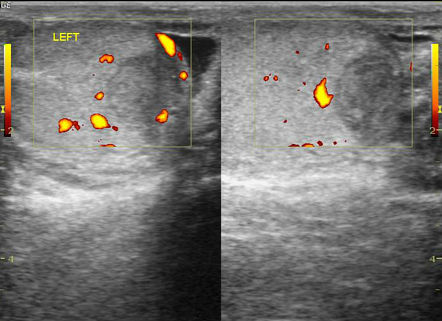This color photograph showcases two side-by-side medical imaging scans, resembling ultrasounds, each framed by bars that gradient from red at the bottom to yellow at the top. The left image features the word "LEFT" in yellow text at the upper left corner. Both images predominantly display grainy white, gray, and black areas, making the specific shapes indistinguishable and forming abstract blobs. At the top of each scan, there's a thin yellow rectangular overlay containing smaller, heat-map-like splotches in yellow and red, suggesting areas of interest. The right image appears to be a zoomed-in view of the left image, offering a closer look at these white blobs and the embedded black blob within the larger white mass.